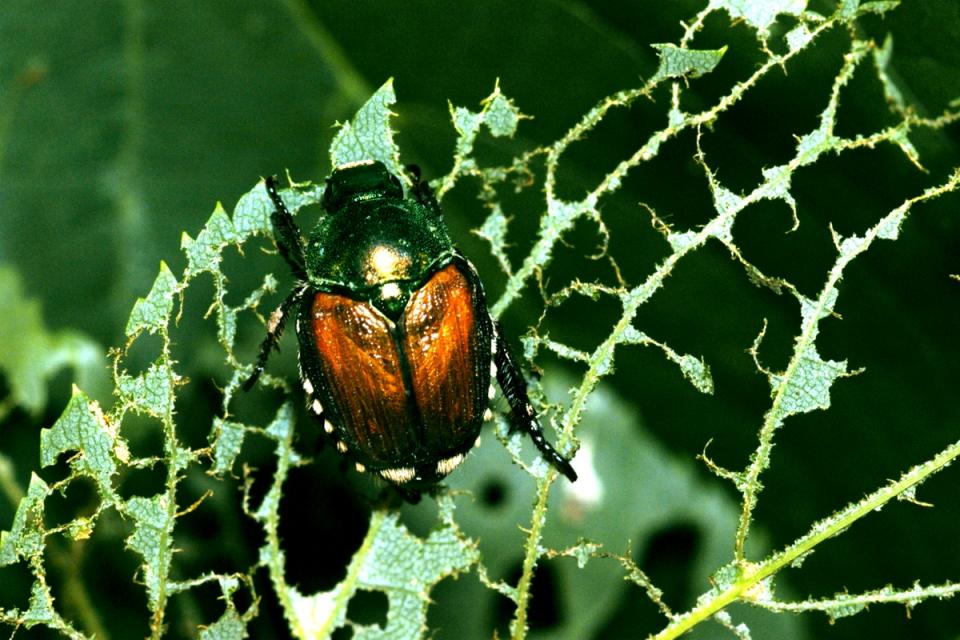A vividly detailed, horizontally oriented color photograph taken outdoors during the day features a large beetle perched on a jagged, chewed-up green leaf. The background is a blurred, lush expanse of big green leaves, amplifying the vividness of the scene. The beetle itself is front and center, sharply in focus, showcasing its distinct features. Its body is robust and dark brown with a hard shell, accented by a line splitting it down the middle and white markings along the edges, hinting at a detailed, almost painterly texture. The head and upper part of the back stand out in a pearl green hue, contrasting strikingly with its black legs, which cling firmly to the green, curved plant stalk. The leaf, visibly damaged with only veins and small sections intact, suggests the beetle is actively feeding. This immersive nature scene captures the intricate beauty and realism of the moment.